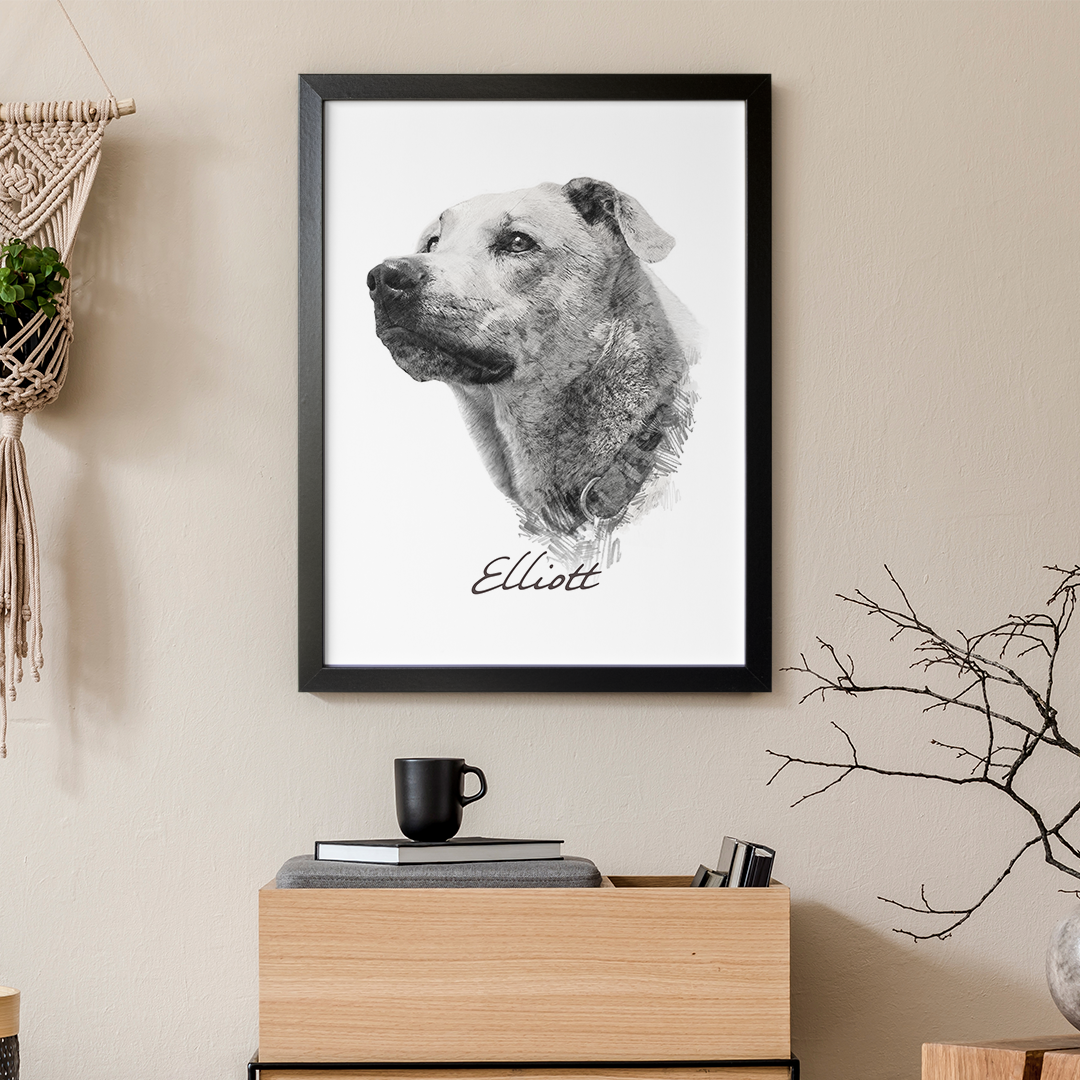The photograph showcases a meticulously arranged room with a Scandinavian, minimalistic aesthetic. The walls are cream-colored, complementing the light tan furniture. The focal point is a prominent charcoal painting of a yellow Labrador, framed in black on a white background, with the name "Elliot" inscribed beneath. This poignant image of the dog, gazing off to the side, appears to memorialize a beloved pet. 

To the left, a macrame flower hanger adds a touch of texture. Below the painting, there's a wooden storage unit with two compartments: the top one containing a blanket, a book, and a black coffee mug, and the bottom one housing several books. On a wooden table to the right, a vase holds a miniature tree, enhancing the room's natural vibe. Despite the cohesive minimalist design, the dog portrait stands out, adding a unique and heartfelt element to the decor.